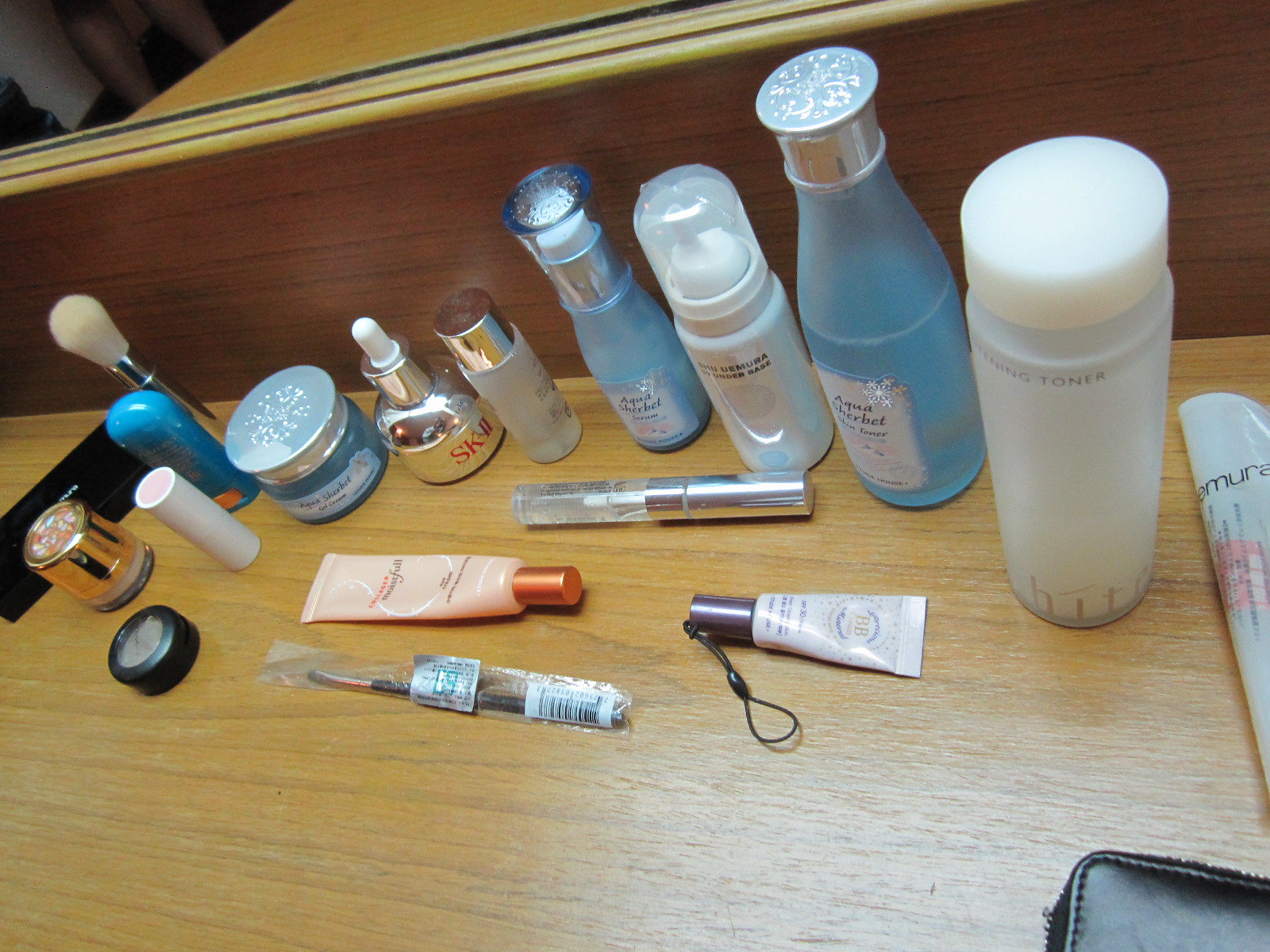A carefully curated collection of beauty products is prominently displayed on a wooden table, likely situated in a bathroom setting. The assortment features between 16 to 19 small bottles, each boasting a variety of colors, including silver, blue, white, and a light orange hue. The bottles, which bear text that is too small to decipher, are meticulously arranged in the center of the image, stretching from left to right. The backdrop reveals a mirror, reinforcing the bathroom environment, and the slightly overhead perspective suggests the photograph was taken by someone standing at the table.